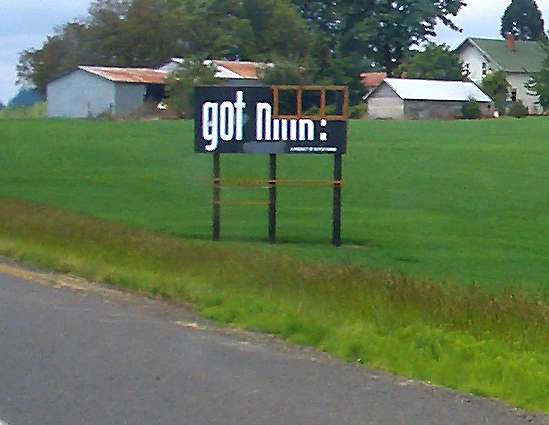The image appears to capture a rural scene featuring a collection of farm buildings against a backdrop of trees and a blue sky. Central to the image is a partially fallen black sign with white text, which seems to originally have said "Got Milk," though it's obscured and incomplete. To the left of the sign, there is an abandoned barn with a rusted metal roof and missing door, indicating neglect and wear. The dilapidated state of the barn contrasts with a white farmhouse nearby, which has a distinctive green roof and red chimney. A third building, constructed from plain wood, also features in the scene. The ground is covered with green grass, and part of an asphalt road with striped markings is visible. The overall quality of the image is poor, likely taken with a low-resolution digital camera.